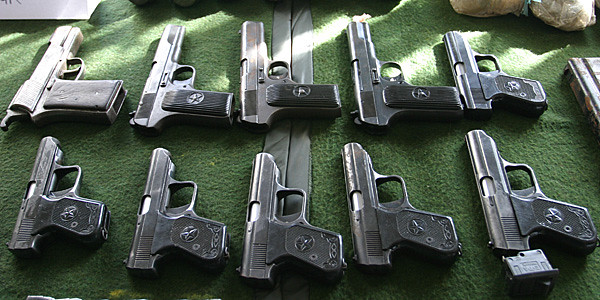In this color landscape photograph, ten handguns are meticulously arranged in two rows of five on a green felt or blanket backdrop. Each gun is positioned flat on its side with the barrels pointing away from the camera and the handles facing to the right. The guns, all exhibiting a dull gray gunmetal color, appear nearly identical except for slight variations in size, particularly in the top row where three or four pistols are noticeably larger than those in the bottom row. The scene is illuminated by sporadic light coming from the upper right, leaving portions of the image in shadow. The handles of the guns show some decorative engravings. Visible in the background, yet partially cut off by the frame, are a small square object on the bottom right, a book or ledger peeking in from the right edge, and additional indiscernible items at the top.